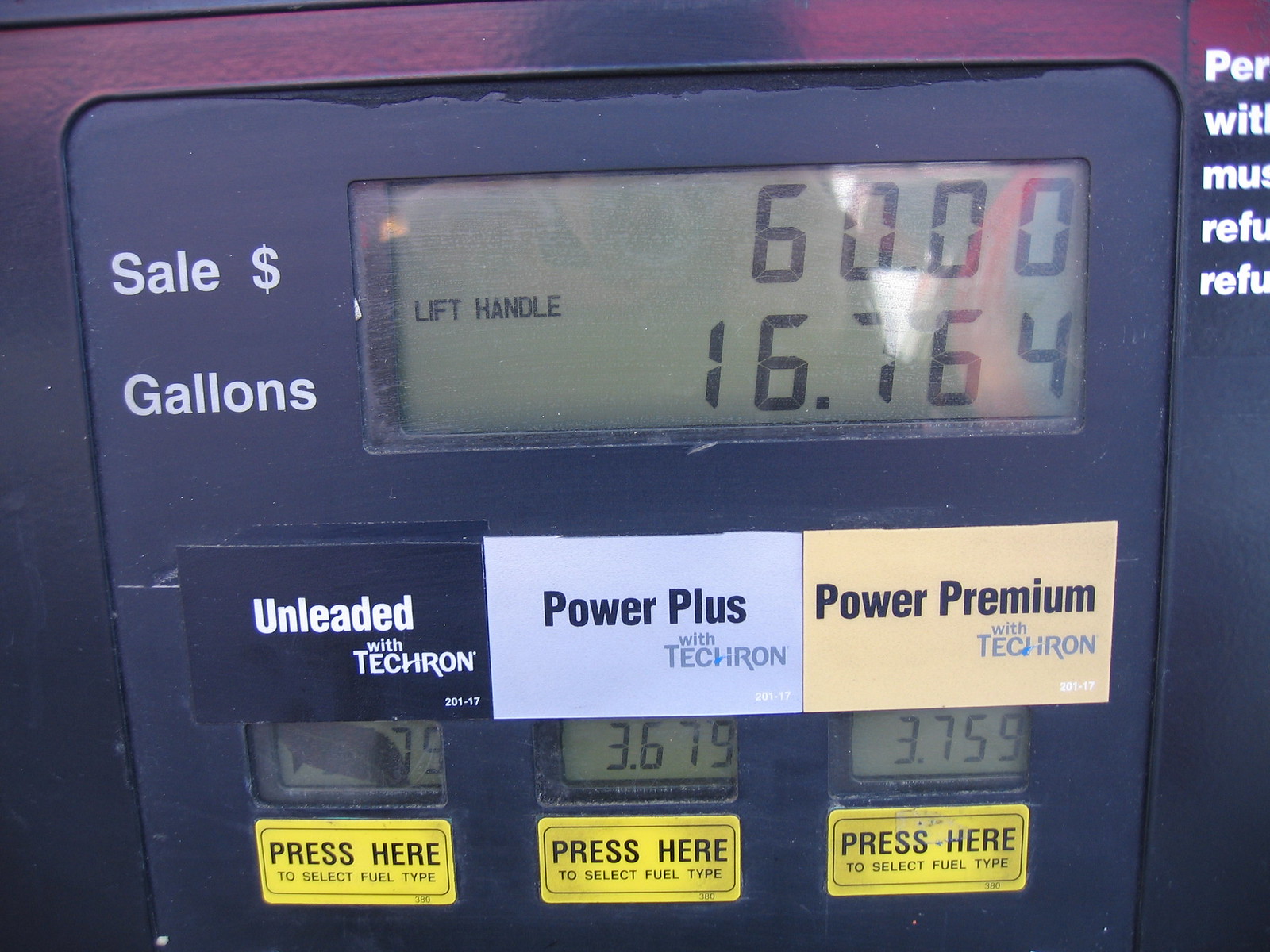The image depicts a weathered black gas pump with a partially chipped or peeling plastic exterior. At the top of the pump is a digital display with a green background and black digital lettering. The display shows a sale price of $60.00 and a total of 16.764 gallons dispensed. To the left of the digital screen are labels in white text indicating "sale" and "gallons," and instructions to "lift handle" are also prompted on the left. Directly below the display, there are three fuel selection buttons: on the left, a black button labeled "Unleaded with Tecron," in the middle, a white button labeled "Power Plus with Tecron," and on the right, a gold button labeled "Power Premium with Tecron." Each button has a small digital display below it showing the price per gallon; "Power Plus" is priced at $3.67 and "Power Premium" at $3.76. Below these buttons, yellow selectors instruct users to "press here to select fuel type." A slight shine or shimmer on the surface of the pump suggests a reflection, adding to the overall visual details of the image.